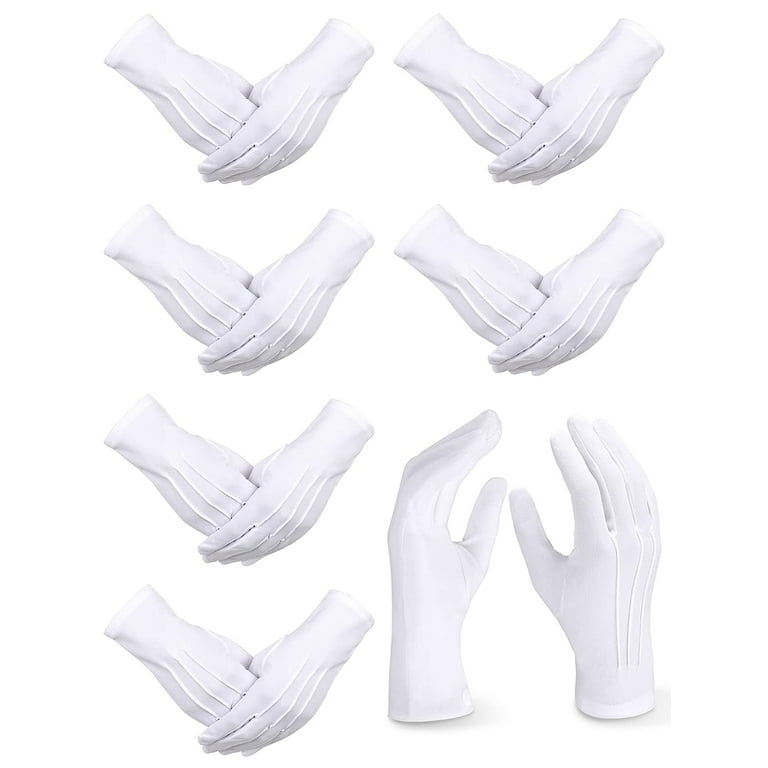The vertically rectangular, monochrome photograph features a series of seven distinct images, divided into a grid-like arrangement with four rows on the left and three on the right. Each of the initial six images displays two white gloves interlocked in a seemingly identical pose, with one glove folded over the other and their thumbs wrapped inside each other. Specifically, the top two rows showcase these intertwined gloves positioned side by side. The left side of the bottom two rows continues this pattern until the third column on the right, where a divergence occurs. Here, the gloves are depicted standing upright, their palms facing outward with one glove slightly rotated away. The minimalistic, white background ensures that the focus remains solely on the detailed, staged positions of the gloves.